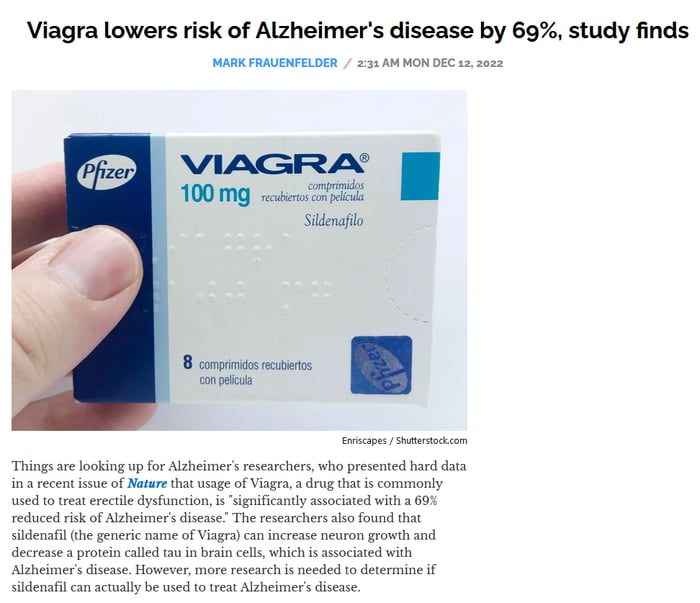**Caption:**

A recent advertisement for Viagra highlights research findings suggesting potential cognitive benefits beyond its primary use. The ad features a close-up image of a man's hand holding a package of Pfizer's trademarked Viagra, 100 mg film-coated tablets, with the packaging text in Spanish: "8 Comprimidos Recubiertos con Película". Beneath the image, black text reads: "Viagra lowers risk of Alzheimer's disease by 69%, study finds" by Mark Frauenfelder, posted on Monday, December 12th, 2022 at 4:31 a.m. The caption mentions photographer Hendrik Escher/Shutterstock.com.

According to a research article published in Nature, Viagra, commonly used to treat erectile dysfunction, shows a significant association with a 69% reduction in the risk of Alzheimer's disease. Additionally, the researchers discovered that sildenafil, Viagra's generic name, promotes neuron growth and reduces tau protein levels in brain cells, which are linked to Alzheimer's. While these findings are promising, further research is needed to confirm sildenafil's potential as a treatment for Alzheimer's disease. The advertisement presents an optimistic outlook for Alzheimer's research, indicating that things may be looking up.